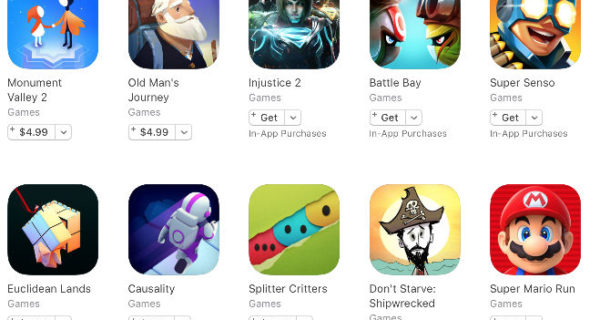The website image displays a vibrant selection of games, each represented by colorful cartoon illustrations. The top row features five games, although the upper portion of each game image is slightly cut off. Despite this, the games remain identifiable. They include Monument Valley 2, Old Man's Journey, Injustice 2, Battle Bay, and Super Cellario. The bottom row showcases Lucadene Lands, Casualty, Splitter Critters, Don't Starve Shipwrecked, and Super Mario Run, with all images fully visible. Notably, Super Mario Run features the iconic Mario against a red background. The first two games on the top row are priced at $4.99, while the remaining three display a "Get" button with a drop-down indicating in-app purchases. Unfortunately, the prices for the games in the bottom row are not visible due to the website layout.